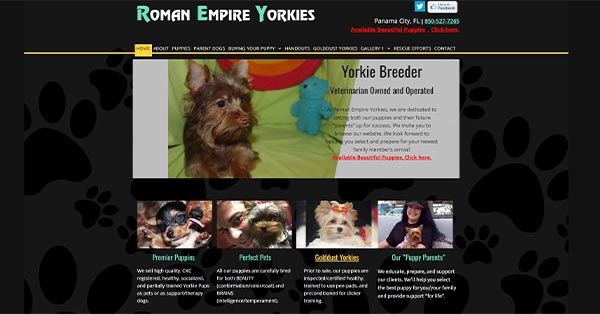Screenshot of the "Roman Empire Yorkies" website in a horizontal, landscape orientation. At the top, the header prominently features "Roman Empire Yorkies" with the letters 'R,' 'E,' and 'Y' capitalized and written in a distinct black or blue font against a white background. The website is identified to be based in Panama City, Florida. Beneath the header, the text "Veterinarian Owned and Operated" is displayed, although some of the smaller text details are unclear and presumably contain information about the breeder's practices and commitment to humane breeding.

Centered in the image is an adorable photograph of a Yorkie puppy. The puppy is comfortably nestled on a pillow, accompanied by a plush stuffed animal and a triple-layered ball spinning toy, evocative of a nurturing and playful environment.

Towards the bottom of the screenshot, four distinct categories are previewed, each with representative images. The categories appear to provide:

1. Information on the Yorkie parents, indicated by the term "Our Puppy Parents" although the exact wording is unclear.
2. Details about specific Yorkie puppies, possibly labeled as "Perfect Pets" or similar, featuring a photograph of a Yorkie with a pink bow, suggesting a focus on female puppies.
3. An unspecified category possibly about the available Yorkies or past litters.
4. Testimonials or photos related to adoptive families and their Yorkies, suggested by the term "Perfect Puppies" or resembling.

Each section emphasizes a photographic representation, likely depicting affectionate scenes of the Yorkshire Terriers and their caretakers, emphasizing the breeder's dedication to their well-being.